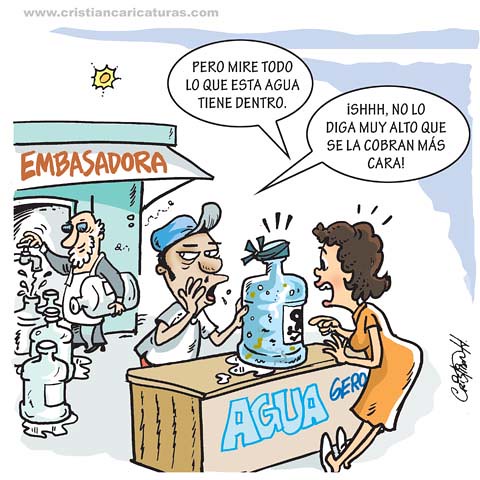The image is a colorful and cartoonish Spanish-language comic strip set outdoors, with a bright blue sky and a small, yellow-orange sun in the top left corner. The top left also has the text "www.christiancaricaturist.com" in gray. The main focus is on a brown table or booth with the word "AGUA" written in light blue letters on a pink background. A large blue jug with a green wrap around its top sits on the booth, appearing to be leaking and dirty. 

On one side of the booth stands a man wearing a blue hat with the bill upturned, and his right hand resting on his cheek. He is making a peculiar expression. Across from him is a woman in a yellow dress, appearing to scream in shock and falling backward while pointing at the jug. Above their heads are Spanish speech bubbles: the woman says, "Pero, mire todo lo que esta agua tiene dentro," while the man replies, "Ay, no lo diga muy alto que se la cobran más cara."

Behind the booth is another storefront labeled "EMBASADORA." An older gentleman with glasses in this area is seen filling jars from a faucet, with several empty jars lined up in front of him. Overall, the scene is a humorous take on a water-selling scenario with exaggerated reactions and expressions.